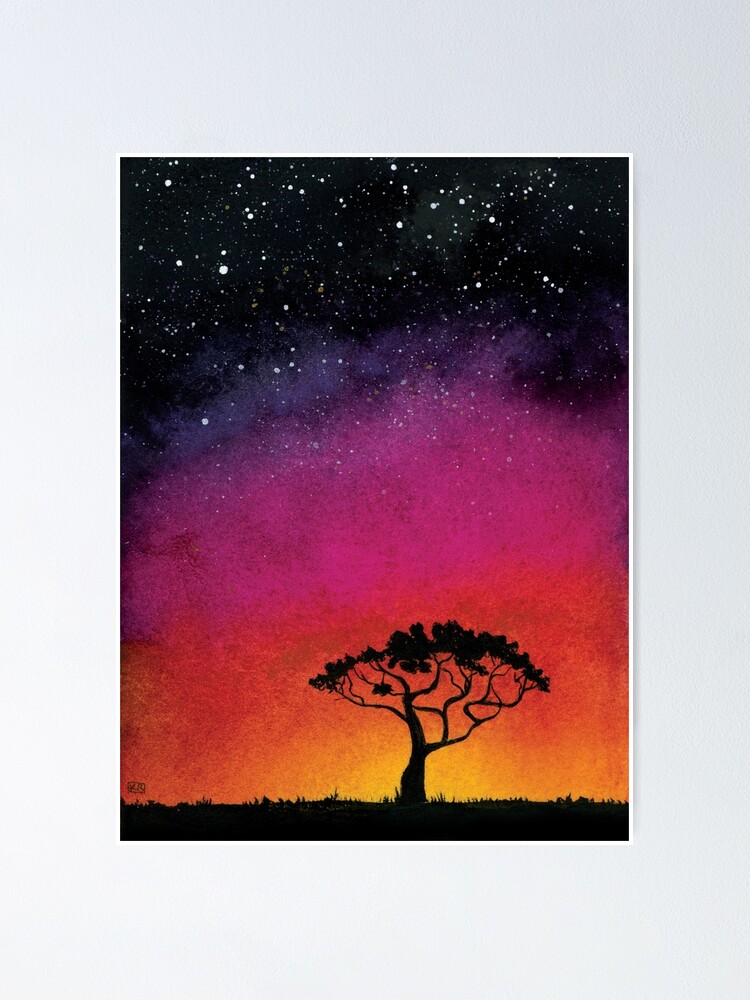The image appears to be a painting or drawing capturing a serene night scene with a vibrant sky. At the center bottom of the image, a lone tree with a wide, arching canopy dominates the scene. The silhouettes of its branches spread in various directions, surrounded by small tufts of grass at the base. The sky behind the tree transitions through a stunning gradient of colors: starting from a warm orange and red hue at the horizon, suggesting the remnants of a sunset or sunrise. This orange seamlessly blends into a mystical purple haze, which further transitions into a deep bluish-black, eventually culminating in a pitch-black sky at the top. The night sky is adorned with countless bright stars, creating a beautiful and clear starry night. The overall composition of the image, with the contrast between the darkened tree and the colorful, starry sky, evokes a dream-like atmosphere, reminiscent of an African wilderness scene.